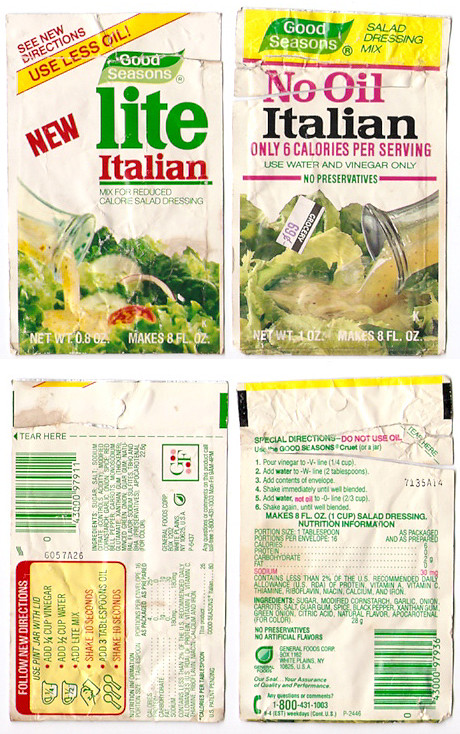The image displays four sauce packets arranged in a grid, with two at the top showing the front labels and two at the bottom revealing the back side of the packets. The top-left packet features a label reading “Light Italian” with the brand "Good Seasons" noted prominently. There's also a "New" tag placed off to the left of the packet. To the right of this packet, the label states "Good Seasons" again, followed by "No Oil Italian." This variety boasts only six calories per serving. Additionally, at the bottom of this packet, there are instructions which say "Follow menu directions or follow new directions."

Focusing now on the back side of the packets, both of which are assumed to be the same "No Oil Italian" variety, the bottom-left packet provides special instructions: "Do not use oil," and provides a serving suggestion that says, "Make six fluid ounces (FLOZ), one cup salad dressing." This arrangement showcases the distinct front and back designs, highlighting the nutritional details and usage instructions for the "Good Seasons No Oil Italian" salad dressing packets.